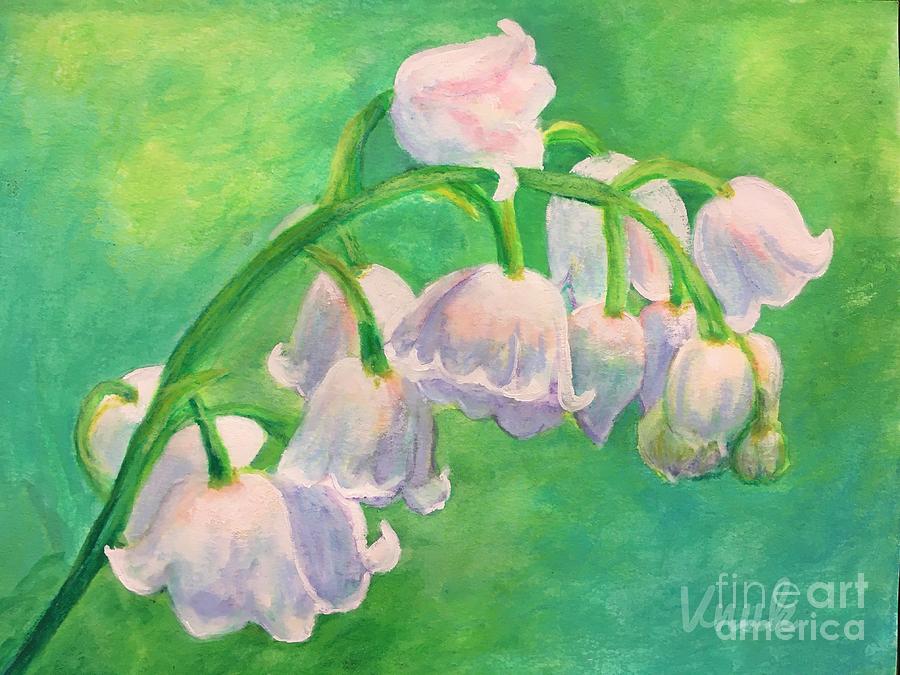This artwork is a meticulously detailed painting of vibrant pink tulip-like flowers set against a rich, green background. The green backdrop features varying hues, with three distinct lighter green spots that gradually converge into deeper shades, giving the composition a dynamic and textured appearance. A green vine gracefully arches through approximately 80% of the canvas, from the lower left moving upwards and slightly rightward, supporting an array of over ten flowers. These flowers, with their delicate pink petals tinged with subtle dark gray shadows, are in different stages of bloom and appear to be wilting, with most of them gently drooping downwards. One flower at the front remains closed, adding variety and depth to the portrayal. The painting's signature, partially obscured by the prominent Fine Art America watermark located in the bottom right corner, hints at the artist's identity while ensuring the work is recognized as part of Fine Art America’s collection. This piece captures the fleeting beauty of the flowers, enhanced by the lush, splotchy green background that envelops the entire scene in a harmonious, natural tapestry.